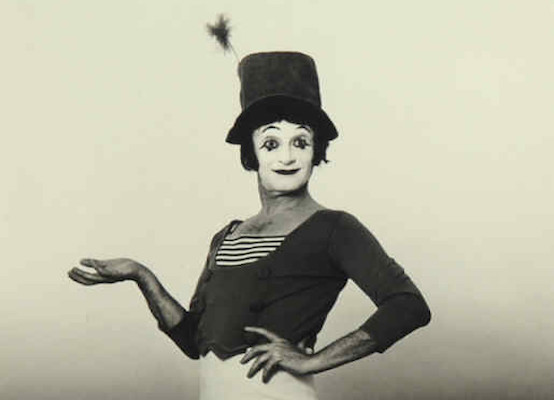In this vintage black-and-white photo, a mime from the early 1900s, possibly between the 1910s and 1920s, strikes a pose against a plain white background with a hint of sepia tone. The mime is slim-bodied and it's likely male, given the presence of some chest hair. Standing with a quizzical smile, he has his left hand on his hip and his right hand raised outward, palm up, as if holding an invisible object. His face is entirely painted white, accented with dramatic black eyeliner and exaggerated black lower lashes, darkened eyebrows, and black lipstick. He wears a tall, floppy top hat adorned with a feather or poof, under which short dark hair peeks out. His attire includes a double-breasted, cropped jacket over a striped tank top, with suspenders and white pants completing his outfit. The mime's enigmatic expression and detailed vintage costume capture the essence of early 20th-century performance art.